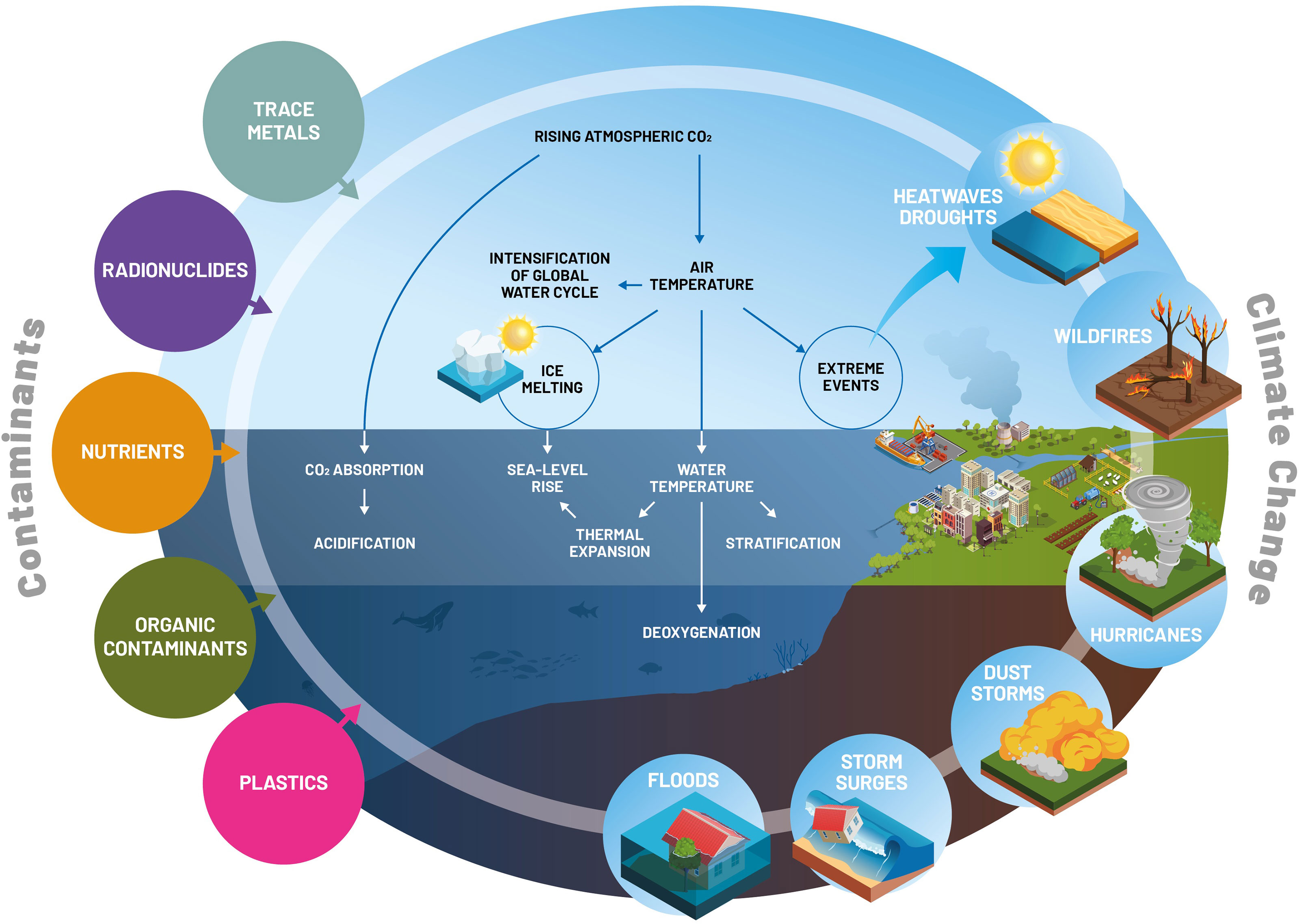This detailed diagram is a colorful illustration of various environmental effects and contaminants on an ecosystem. The main feature is a large, centrally positioned oval shaded in three gradient colors representing different layers: light blue for the sky at the top, a bluish-gray for the water in the middle, and transitioning to dark blue and brown for the underwater ground at the bottom. On the right middle, a green landmass with buildings signifies a populated area.

On the left side of the oval, several multicolored circles with white, all-caps text encircle the main diagram. Starting from the top, a green circle labeled "TRACE METALS" has an arrow pointing to the sky. Below it, a purple circle marked "RADIONUCLIDES" has another arrow targeting a different sky section. The light brown circle labeled "NUTRIENTS" points to the just-underwater section, while a dark green circle labeled "ORGANIC CONTAMINANTS" targets a deeper underwater section. At the bottom, a dark pink circle labeled "PLASTICS" also points to an underwater area. This array of circles is collectively labeled "CONTAMINANTS," vertically written in gray letters.

On the right side, another set of circles, each depicting different climate change phenomena, follows the curvature of the oval from bottom to top. These include terms like "FLOODS," "STORM SURGES," "DUST STORMS," "HURRICANES," "WILDFIRES," "HEAT WAVES," and "DROUGHTS" in white text. Above these, significant climate change effects such as "HEAT WAVES," "EXTREME EVENTS," "SEA LEVEL RISE," and "RISING ATMOSPHERIC CO2" are highlighted, pointing towards various sections within the diagram.

Collectively labeled as "CLIMATE CHANGE" in vertical gray lettering on the right, these elements provide a comprehensive view of how contaminants and climatic shifts interact with and impact an ecological system.